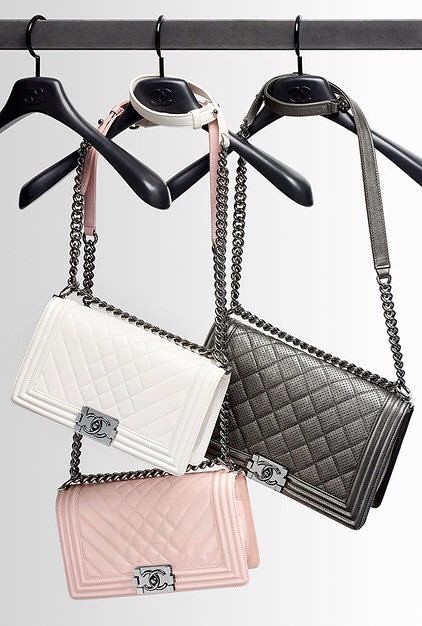This image captures an indoor scene with a white background, likely taken inside a closet. Displayed prominently in the photograph is a rectangular, dark-grey clothes rod without an additional crossbar at the bottom. Three thick, black plastic hangers with metal hooks hang from the rod. The leftmost hanger is empty.

The center hanger holds two purses—one white and one pink. Both purses feature a distinctive design: a diamond-shaped pattern on their surfaces and a metal clasp in the center with a decorative logo of two intertwined 'C's. The purses are identical in style with chain-link straps that transition to a matching leather section for over-the-shoulder wear.

The hanger on the right showcases a slightly larger gray purse with the same diamond pattern and logo. Similar to the other purses, it has a chain-link strap with a leather section at the top. The purses hang securely from their respective hangers by wrapping the leather part of the straps around the thickest part of the hangers.

Overall, this image is a detailed showcase of three elegant purses, organized and displayed for visual appeal, emphasizing their uniform design and color variations.